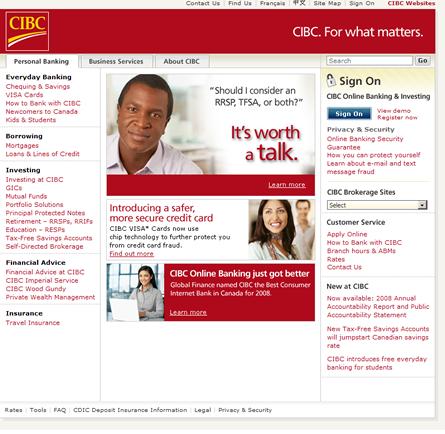The image features a website header with a CIBC logo prominently displayed in the upper left corner. The logo consists of yellow font set against a red background, with a red strip beneath it stating the slogan "CIBC for what matters." To the right of the logo, and starting from the middle of the image, a series of web navigation links are listed, including "Contact Us," "Find Us," "France," "Kanji," "Site Map," "Site On," "CIBC Websites," and "ES." Although some text appears blurred due to poor resolution, these elements are distinguishable.

Further down the header, a set of navigational tabs is aligned to the left, labeled "Personal Banking," "Business Services," and "About CIBC." Opposite these tabs, on the right side of the header, there is a search bar with an accompanying "Go" button.

Beneath the header, the left-justified menu showcases a range of services under different categories. The first category, "Everyday Banking," is highlighted in black, followed by links in red text: "Checking and Savings," "Visa Card," "How to Bank with CIBC," "Newcomers to Canada," and "Kids and Students."

A horizontal line separates this section from the next category, "Borrowing," also in black. The associated links in red text include "Mortgages" and "Loans and Lines of Credit." 

Further down, another grey line delineates the final category, "Investing," written in black, with red text links for "Investing at CIBC," "GICs," "Mutual Funds," "Portfolio Solutions," "Principal Protected Notes," "Retirement," "RRSPs," "RRIFs," "Education," "RESPs," "Tax-Free Savings Accounts," and "Self-Directed Brokerage."